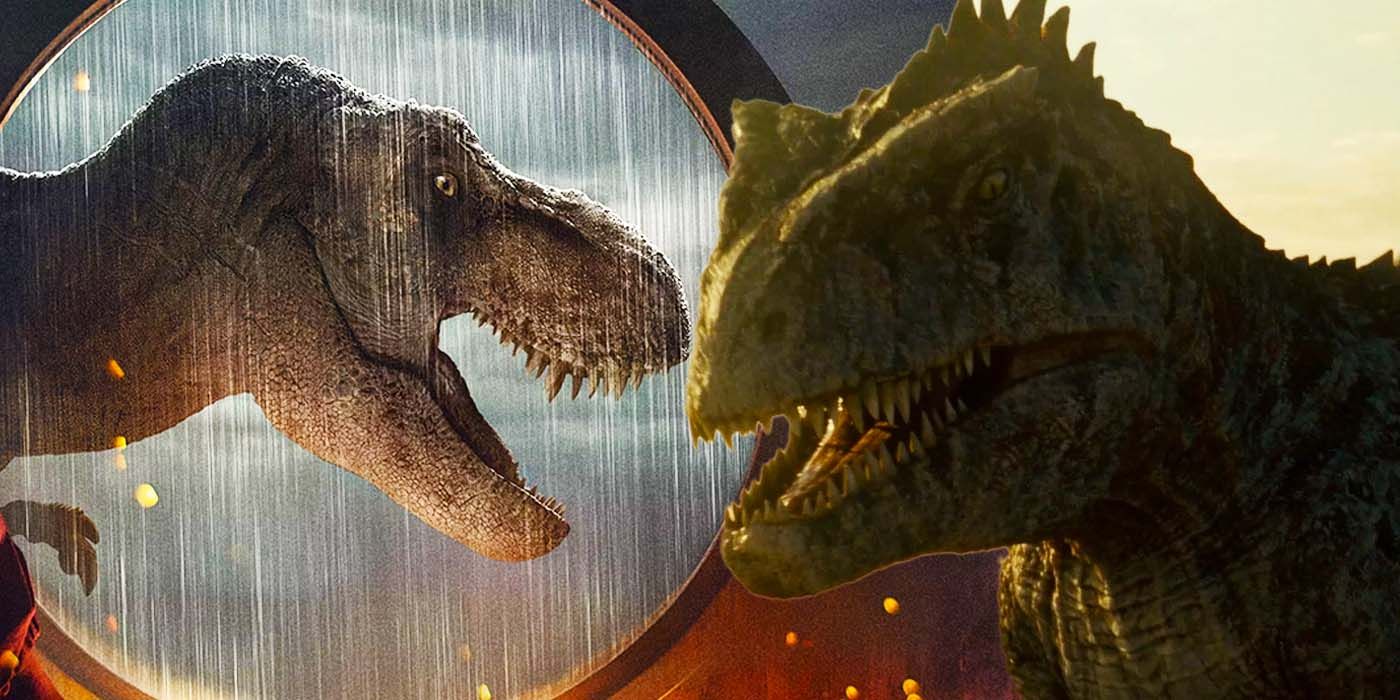In this detailed image, likely a still from a movie or TV show reminiscent of Jurassic Park, we see two menacing dinosaurs facing each other. On the left side of the image, the head and neck of a grey T-Rex are framed by a circular window with a copper border, through which heavy rain is pouring down. This dinosaur is depicted in a complete side view with details such as its roaring mouth and possibly one of its hands visible. The right side of the image features a slightly larger, dark green dinosaur with a more pronounced V-shaped head and sharp teeth. This dinosaur, shown from a diagonal viewpoint, seems to be submerged in a tense atmosphere under a bright sky in the upper right corner. The two dinosaurs create a dramatic tension as they face each other, with the scene carefully crafted to make the image appear cohesive and intense.